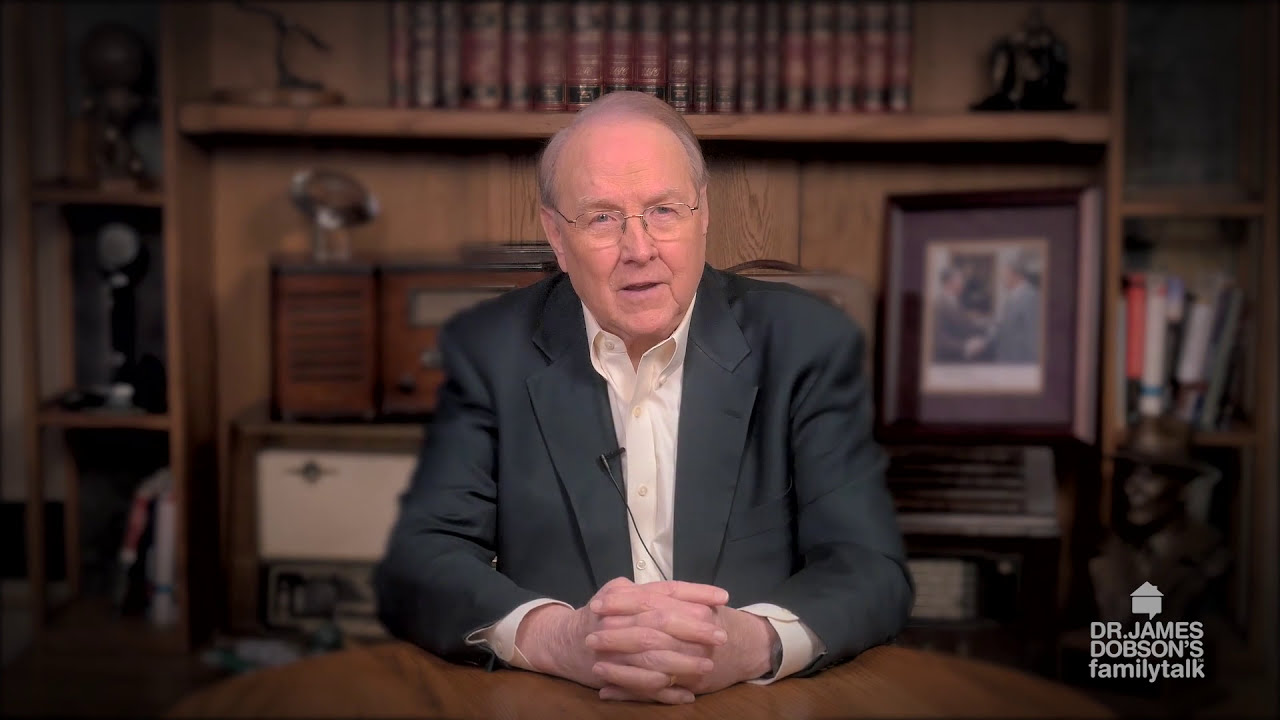The image is a still frame from a video featuring Dr. James Dobson, a politically conservative commentator, as identified by the white text in the bottom right that reads "Dr. James Dobson's Family Talk," accompanied by a two-dimensional house logo. Seated at a circular wooden table with his hands folded, Dr. Dobson, an elderly white man likely in his early 70s, is centrally positioned and facing the camera. He is dressed in a dark gray or charcoal blazer over a white button-down shirt, with no tie. A lapel microphone is clipped to his jacket. He has balding gray hair and is wearing glasses, appearing to speak mid-sentence. The background features a blurred bookcase containing various items such as books, an old radio set, and several trophies or statues. There's a framed photograph of two people shaking hands and possibly an encyclopedia at the top. The setting appears to be a study or office, providing a formal yet scholarly ambiance to the scene.